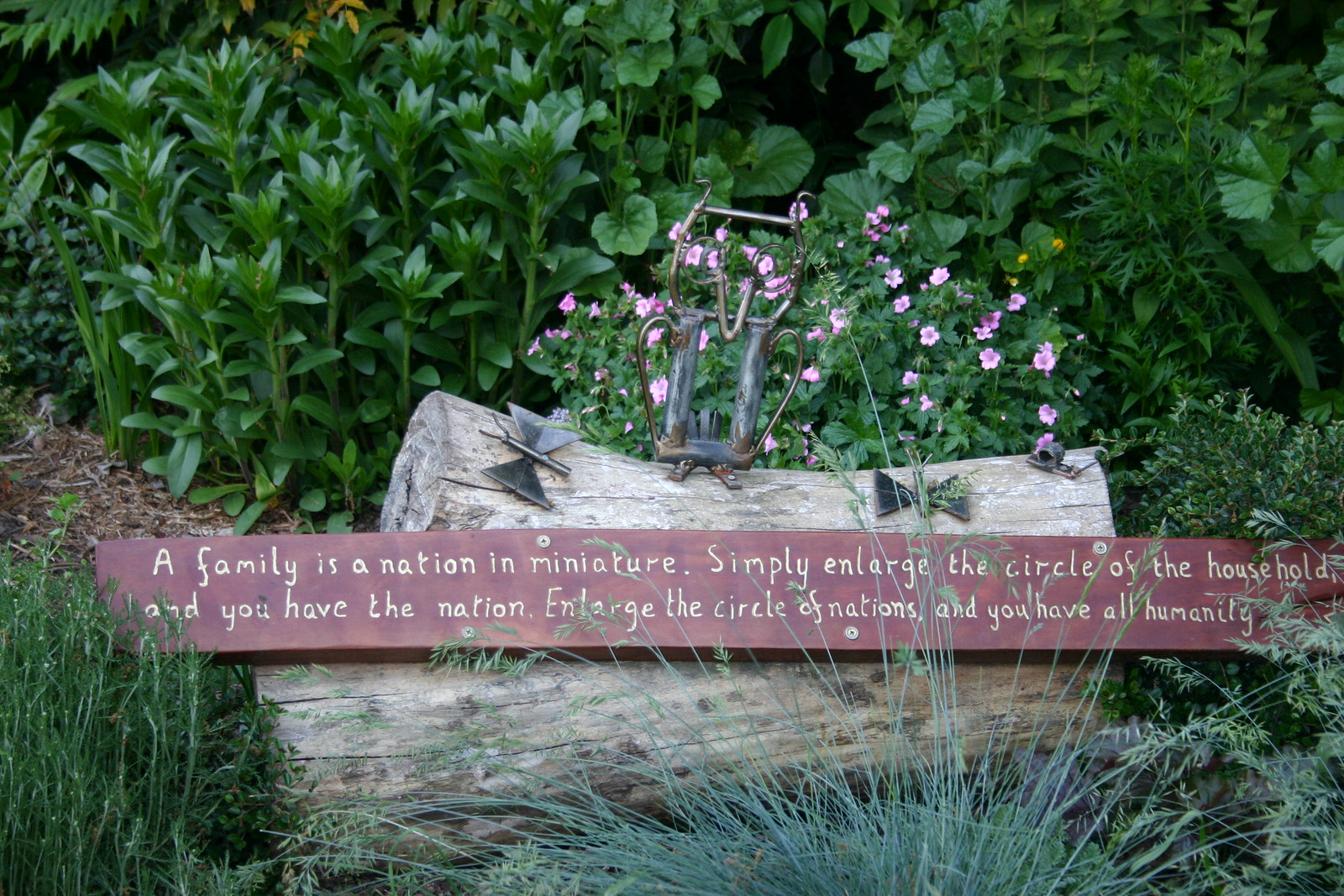This color photograph captures a serene garden scene showcasing a commemorative arrangement with intricate details. Central to the image is a dark brown, wooden plaque, roughly the size of a 2x4, bearing an engraved inscription in yellow that reads: "A family is a nation in miniature. Simply enlarge the circle of the household and you have the nation. Enlarge the circle of nations and you have all humanity." This plaque is securely mounted on an aged, gray log, which is surrounded by lush greenery and light green grass at the front, while brown mulch lines the background. Notably, situated on the log are two steel sculptures of butterflies, with spread wings and delicate antennae. Between them sits an owl sculpture, crafted from thin steel, showcasing intricately bent wings and prominent ears. Behind the log, purple flowers and tall green plants further enrich the scene, adding to its tranquil and reflective ambiance.